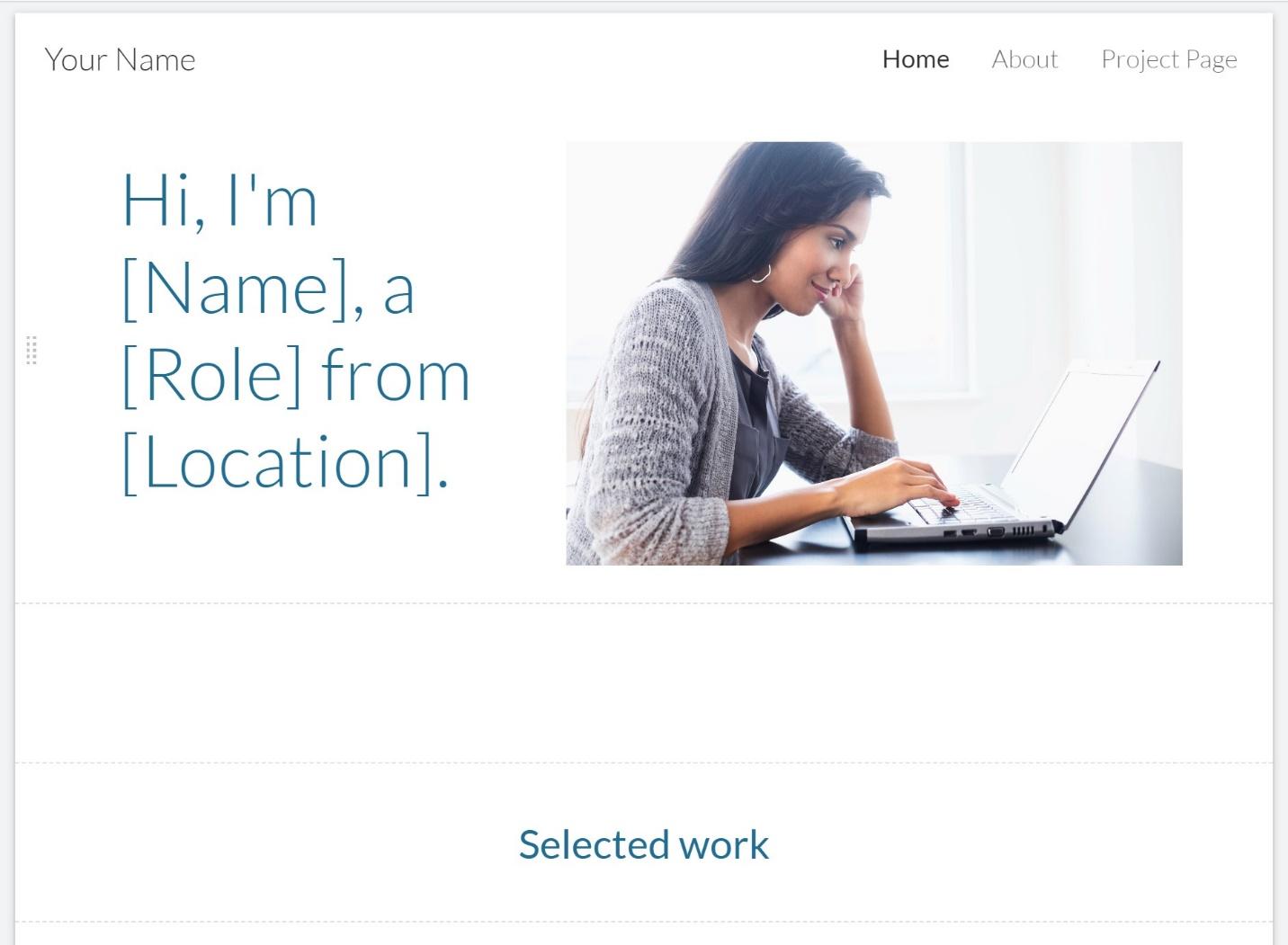**Detailed Caption:**

This is a screenshot of a desktop application interface. In the upper left-hand corner, the user's name is displayed prominently. The upper right-hand corner features navigation options including "Home," "About," and "Product Page." The "Home" tab is highlighted in black, indicating it is currently selected, while the other tabs are grayed out.

Below the navigation bar, the left side of the screen displays a large teal font greeting, which reads "Hi, [Name]" with placeholders for the user's name, role, and location in parentheses. This area allows for customization based on the user's details.

On the right side of the screen is an image of a young woman, possibly in her twenties, with a medium skin tone that suggests an Italian or Mediterranean background. She has long black hair flowing past her shoulders and is dressed in a light grayish-white sweater with sleeves rolled up to her elbows. She also wears a gray shirt underneath and silver hoop earrings. The woman is seated at a desk, looking down with a closed-lip smile. Her left hand rests on her chin, supported by her elbow on the table, while her right hand is placed on a keyboard. Bright light shines behind her, adding a warm glow to the scene.

Centered below her image is the section title "Selected Work" in teal font. This heading is separated from other sections by gray horizontal lines above and below, which help to delineate this particular area of the interface.